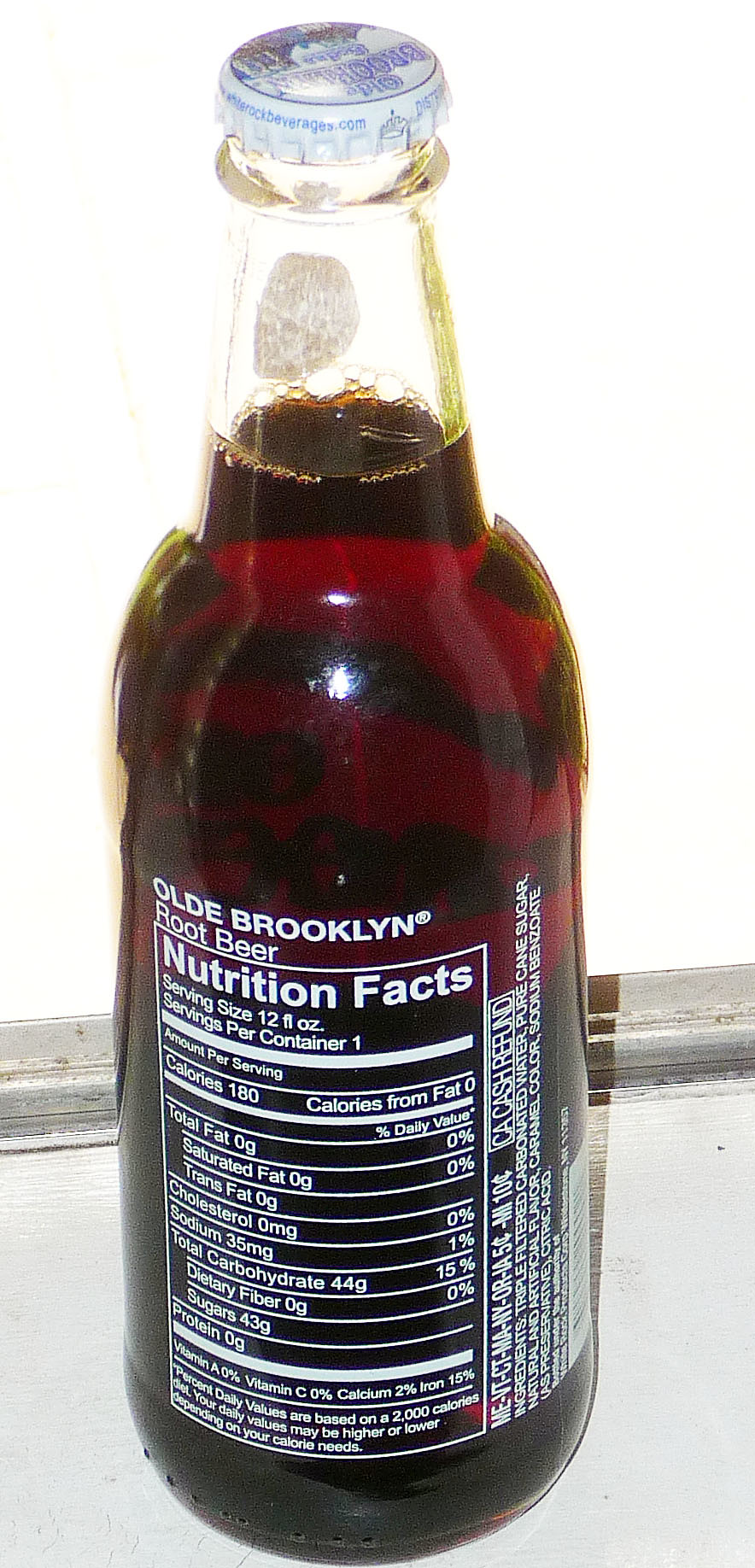In this vertically oriented rectangular image, we see a photograph of a vintage-style glass bottle of root beer, reminiscent of classic brands like A&W or Stewart's. The dark brown root beer inside the bottle contrasts sharply with the light-colored background, as it rests atop a white table or counter. The focal point is the back label of the bottle, which reads "Old Brooklyn Root Beer" in white print. Below this branding, a detailed nutritional information panel is displayed within a rectangular box. The label specifies the serving size as 12 fluid ounces, with 1 serving per container. It lists the contents as 180 calories, with zero calories from fat. The sodium content is 35 milligrams, total carbohydrates are 44 grams, and sugars constitute 43 grams, while protein is absent at 0 grams. At the bottom, a note states that the percent daily values are based on a 2,000-calorie diet. To the right of the nutrition information, the text runs vertically, indicating a "Cash refund in California." The ingredients are also listed, including triple filtered carbonated water, pure cane sugar, natural and artificial flavor, caramel color, and sodium benzoate.